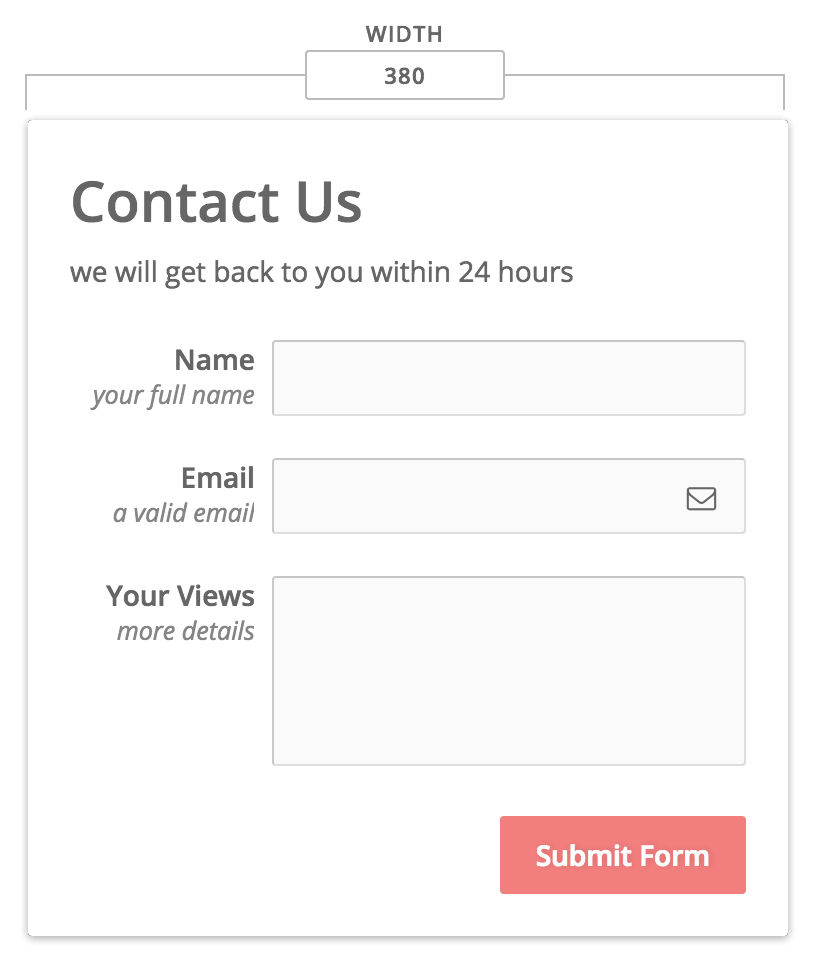The image showcases a screenshot of a basic "Contact Us" template designed for a web page. At the top of a white box, the title "Contact Us" is prominently displayed in enlarged, dark text. Beneath this title, there is a brief statement that reads, "We will get back to you within 24 hours."

Following this, there are several input fields arranged vertically for users to fill out their details. The first field is labeled "Name" in dark letters, with placeholder text below it in gray that says "Your Full Name." This input field is currently blank.

The second field is labeled "Email" and has lighter placeholder text that reads "A valid email." This field is also empty. Adjacent to this field, on the right, there is a small envelope icon.

The third input field, larger than the previous two, is labeled "Your Views" in dark text, with placeholder text below it that says "More details." This field is awaiting user input.

At the bottom of the input fields, there is a prominent red button with white text that states "Submit Form."

Above the "Contact Us" box, there is a smaller section that contains the title "Width" and a field box displaying the number "380." Lines extend from either side of this value to the edges of the "Contact Us" box, indicating that the designated width for this component on the web page is set to 380 pixels.